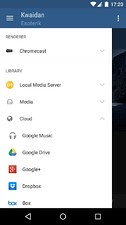This image displays a screenshot taken from a smartphone. At the top, a blue banner is visible, alongside various status icons. On the upper right corner, icons indicating Wi-Fi connectivity, battery level, and the current time are displayed in white. The primary background of the screen is predominantly white. At the very top, there's a line of text which is too small to read, followed by another line of similarly illegible text. Below these, there are several more lines of text accompanied by icons on the left side. Among these icons, a headphone icon indicating audio files, a blue icon representing images, and a folder icon for downloads are discernible. Overall, the image is very small, making the text difficult to read and the details challenging to discern.